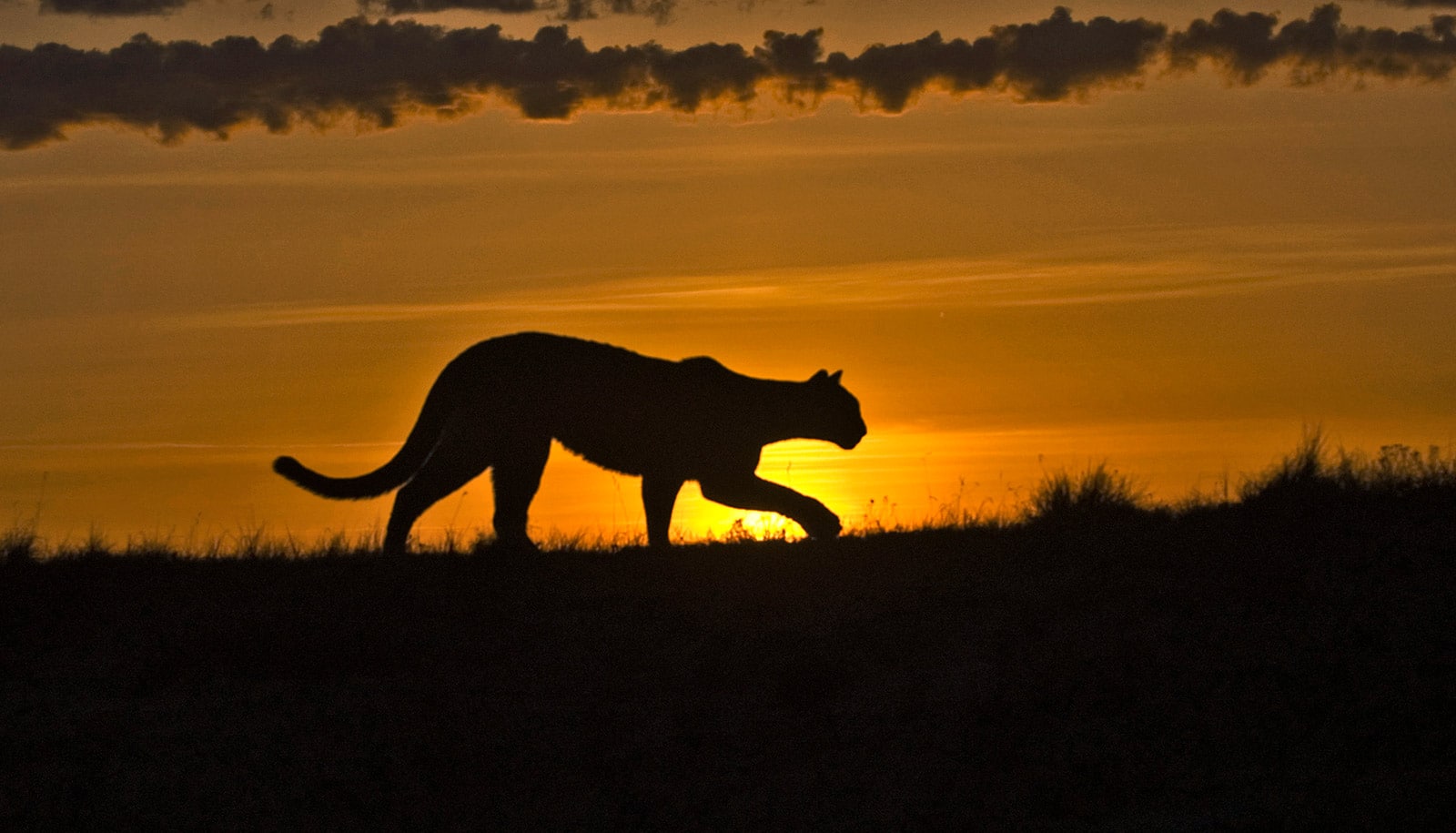The image depicts a silhouetted wild cat, likely a lion or tiger, walking across the dark grasslands during an African sunset. The sky is ablaze with golden hues, streaked with vibrant orange and yellow from the setting sun. Below the cat's head, the bright sun begins to dip below the horizon, casting long shadows. The cat appears intent and deliberate, with its head slightly down and tail curled downward. Its triangular ears and crouching posture suggest that it is moving quietly and cautiously. Above, the sky is adorned with a blend of puffy clouds in a straight line interspersed with thin, wispy clouds resembling contrails. The top of the image is framed by these clouds against a backdrop of a rich, colorful sunset, enhancing the dramatic silhouette of the solitary predator.